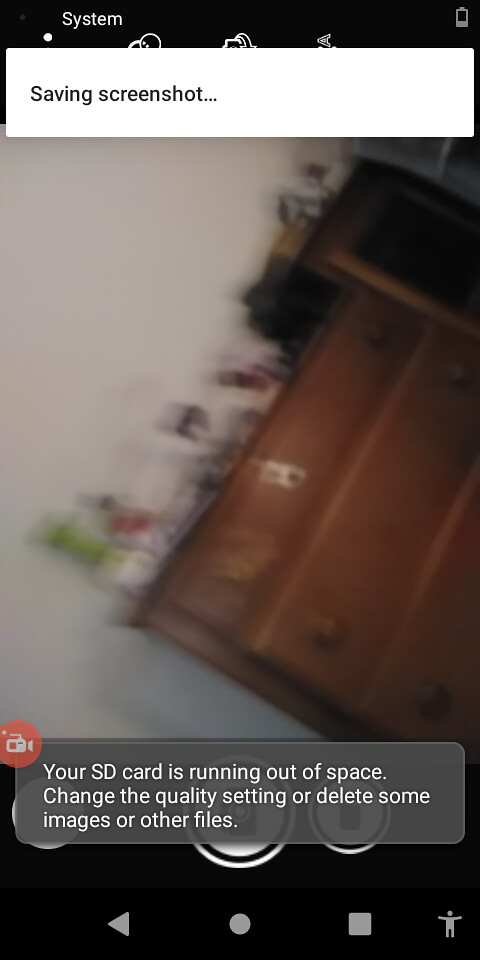The image captures the user interface of a device taking a screenshot. At the top, there's a white notification box with the text "Saving screenshot" in black. Above this box, a black strip labeled "System" in white text is visible. Partially obstructed by the white box are small images or icons.

In the top right corner, the battery icon shows a low charge. At the bottom, within a translucent gray box, there's a red circle with a white camera icon on the top left. The notification in this box reads: "Your SD card is running out of space. Change the quality setting or delete some images or other files."

Behind this translucent box, a black area displays several white buttons, though these are obscured and difficult to identify. Below this interface area are icons including a gray circle, a left-pointing triangle, a square, and a small person symbol in the bottom right.